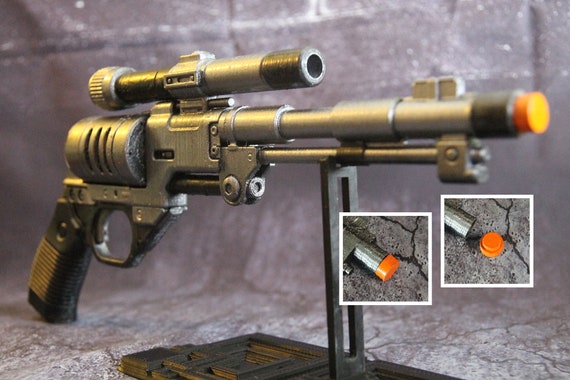The image depicts a detailed model gun with a distinctly steampunk aesthetic. The weapon, which is clearly identified as a model by the orange tip, indicating it is a fake or toy, is primarily silver with a variety of intricate parts not typically found on a standard handgun. The gun features a black pistol grip and a long silver barrel with engraved marks. It is equipped with a prominent silver scope mounted on top, supported by a black rod or rectangular base. The entire assembly is displayed on a wooden and black metal stand. The backdrop appears to be a textured wall resembling scratched stone or metal, further enhancing the steampunk vibe. Additionally, the image includes two smaller inset pictures focusing on the front of the gun, illustrating the difference with and without the orange end cap. The overall design suggests influences from video games, possibly resembling weaponry from titles like Fallout 4.